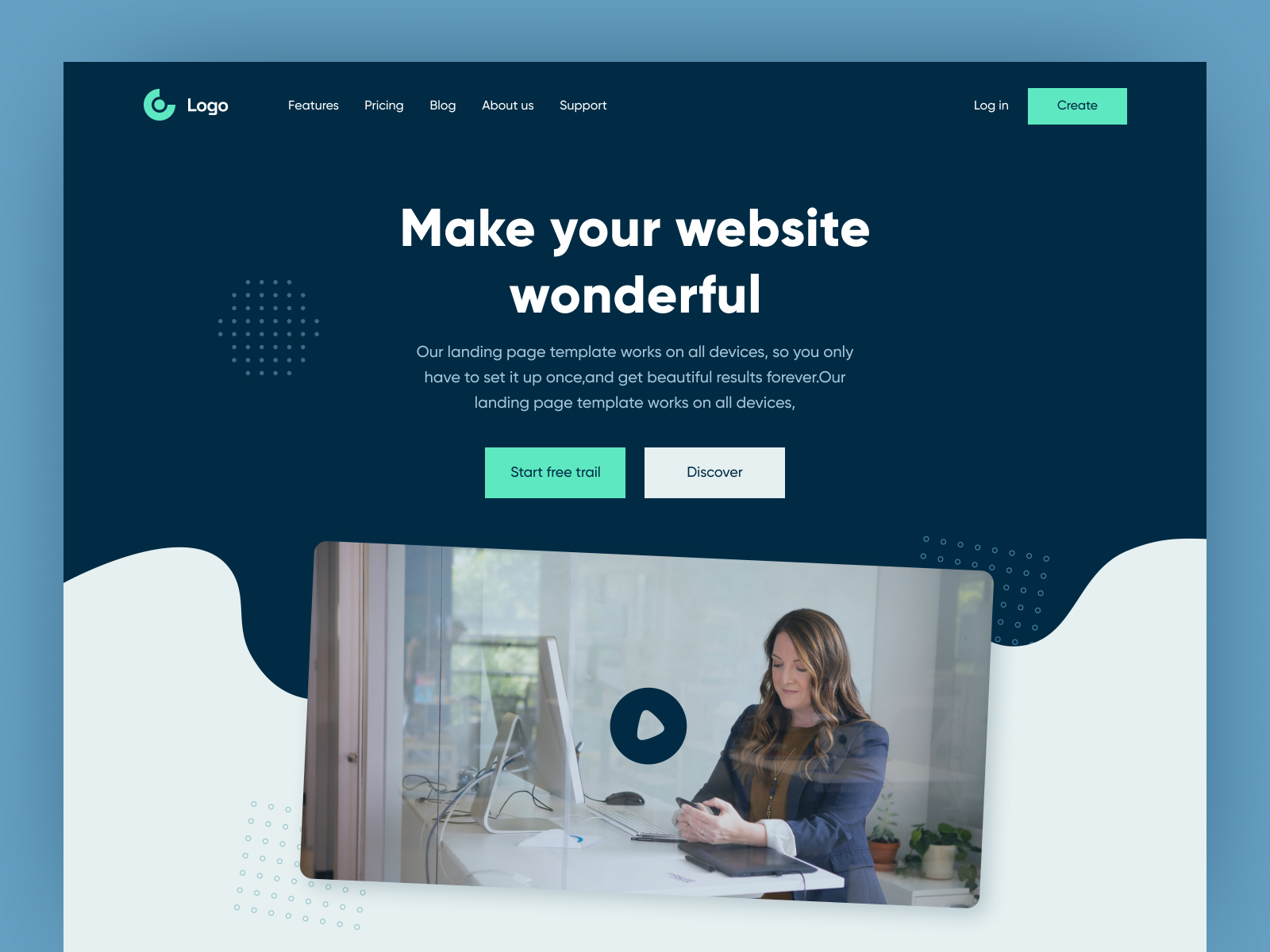In the image, the top left corner displays a logo accompanied by a circular emblem in a greenish-blue hue. Adjacent to the logo, several categories are listed, including "Features," "Pricing," "Blog," "About Us," and "Support." On the top right, two more categories appear: "Create" and "Log In." Notably, the "Create" button shares the same greenish-blue background color as the logo.

Centrally positioned in bold text are the words "Make Your Website Wonderful," with a subheading below in a slightly smaller font stating, "Our landing page template works on all devices. Set it up once and get beautiful results forever." Directly beneath this text are two boxed buttons: the left one reads "Start Free Trial" and is highlighted in the same greenish-blue color, while the right one reads "Discover" and remains white.

At the bottom of the image is a rectangular video frame featuring a woman with brown hair and fair skin, dressed in a blue jacket, looking at her phone. This video element adds a dynamic and engaging visual to the entire design.